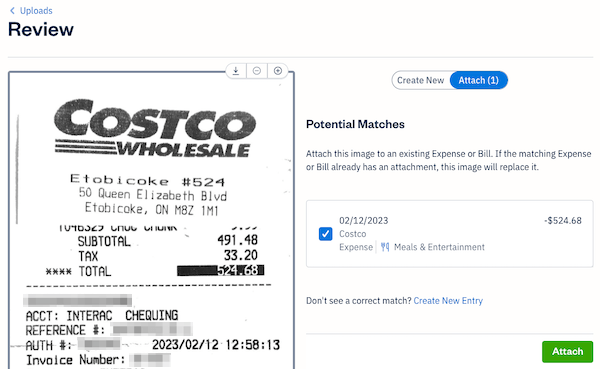In the upper left-hand corner of the image, the word "Uploads" is displayed in a very small blue font, accompanied by a back arrow to its left. Beneath "Uploads," the word "Review" appears in a larger, bolder black font with a capital "R." 

A grey separator bar divides this area from the content below. The page is divided into two sections: left and right. On the left, there is an uploaded image of a receipt from Costco Wholesale, specifically from the Etobicoke location in Ontario, with the store number 524. The receipt details a total amount of $524.68.

On the right section of the page, there is an option labeled "Attach," with a check mark next to the text "Costco $524.68," indicating the receipt has been successfully attached or selected.